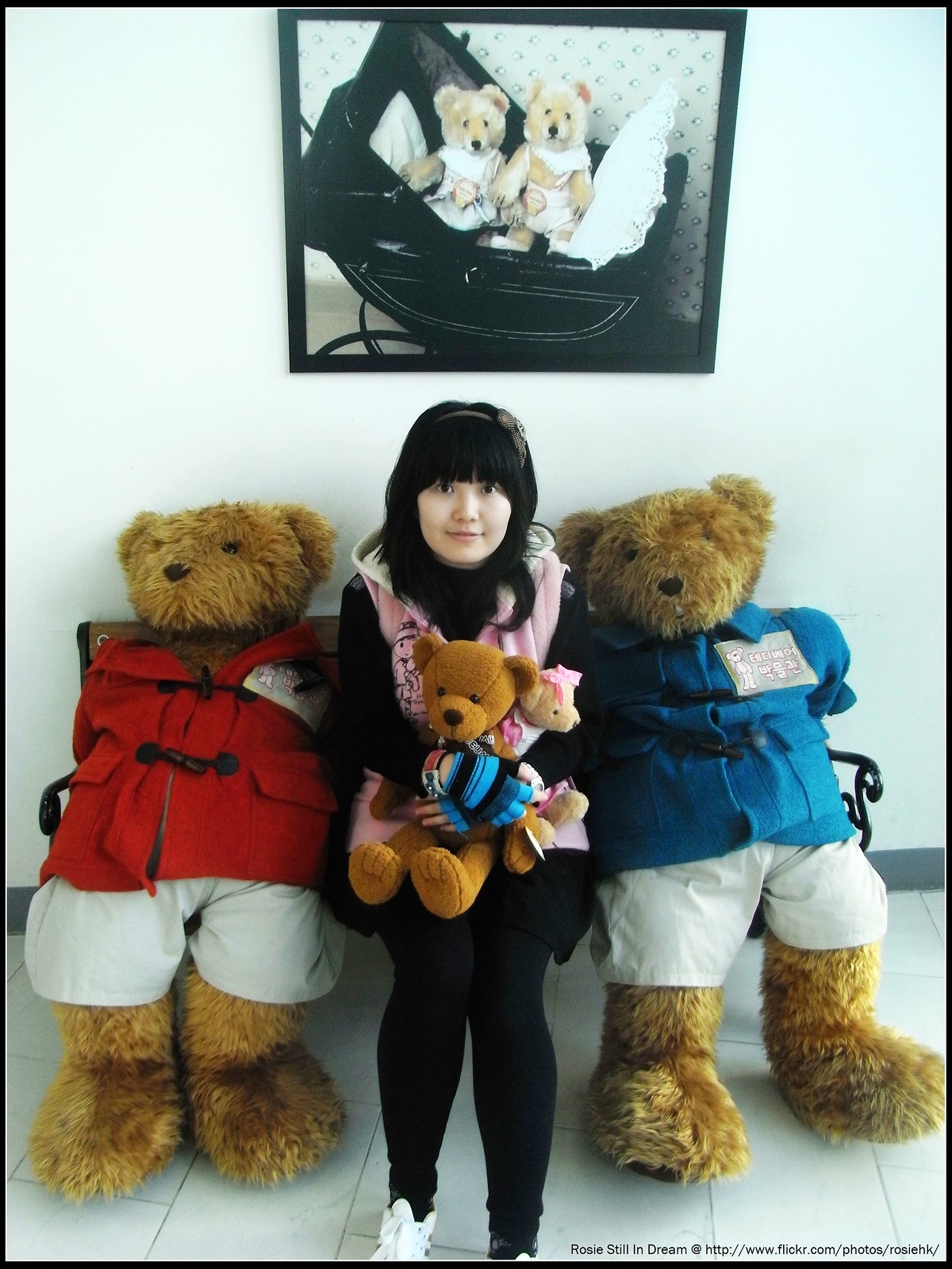In the image, an Asian girl with black hair and wearing a headband sits on a black bench between two life-sized, light brown teddy bears. She is wearing black pants, a black jacket, a pink vest, blue gloves, and white shoes. The girl is holding two teddy bears: one medium-sized and one smaller. The large teddy bear on her left is dressed in a red jacket with toggles and white shorts, while the one on her right is in a blue toggle jacket with white shorts. Each jacket has a patch on the left side. Above the girl is a picture mounted on a white wall, featuring two teddy bears in a black, old-fashioned baby carriage with white pillows on either side of them. The floor beneath them is white tile, complementing the serene setting. The girl gazes directly at the camera, adding a touch of warmth and engagement to the scene.